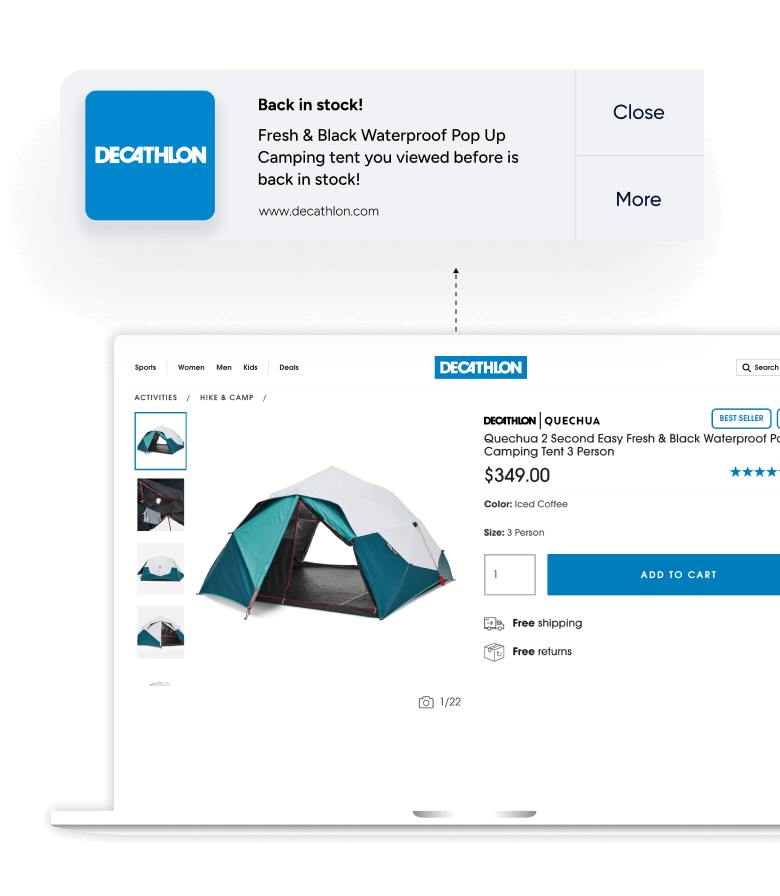This image captures a detailed webpage from Decathlon's online store. At the top of the screen, there is a rectangular banner featuring the "Decathlon" logo in white text set against a blue square background. Below this banner, there's an announcement highlighted with "Back in Stock!" and it informs the viewer that the "Fresh & Black Waterproof Pop-Up Camping Tent" they previously viewed is now available again. The website is identified as Decathlon.com, and users are given options to "Close" or learn "More" about the product.

Scrolling down, the main focus shifts to the tent itself. The product displayed is the "Quechua 2 Seconds Easy Fresh & Black Waterproof Pro Camping Tent" for three people. The brand names "Decathlon" and "Quechua" (spelled Q-U-E-C-H-U-A) are prominently mentioned. This tent is labeled as a best seller and has a rating of four stars, although it's unclear if the rating is out of five stars due to the cutoff. The price of the tent is listed as $349.

The tent color is "Iced Coffee," and its size is specified to accommodate three persons. There is a visible "Add to Cart" button, indicating that the product comes with free shipping and free returns. Additionally, the main image of the tent is displayed prominently, with four smaller thumbnail images on the left side for a better view of different angles or features of the tent.